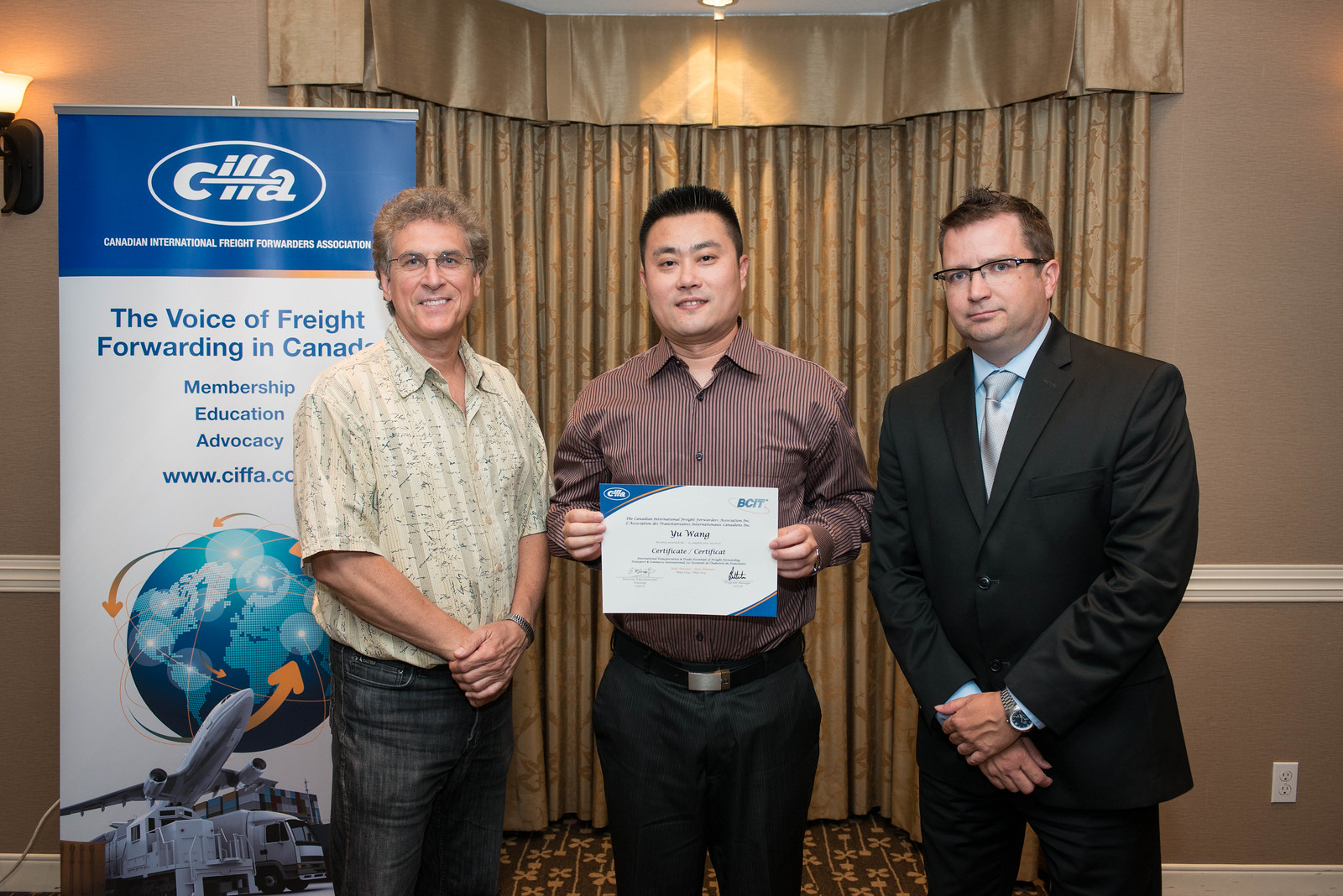In the photograph, three men are positioned side by side, each projecting a serious demeanor. The man on the left is holding a certificate and wears a formal black suit paired with a blue shirt underneath. The central figure dons a red striped shirt and has curly hair, while the man on the right wears a crisp white shirt and glasses, with dark hair neatly styled. In the background, partially opened curtains frame the scene, providing a stage-like setting. 

Above the men is a bold inscription that reads "Scylla, the Voice of Freight Forwarding in Canada," signifying their association with the logistics industry. A prominent graphic of a globe, an airplane, and an arrow pointing forward underscores the international and dynamic nature of their work. The men appear to be poised, their hands either folded or, in the case of the certificate-holder, extended to display the document. The overall composition of the image conveys a sense of formality and purpose, emphasizing the significance of their roles in freight forwarding.